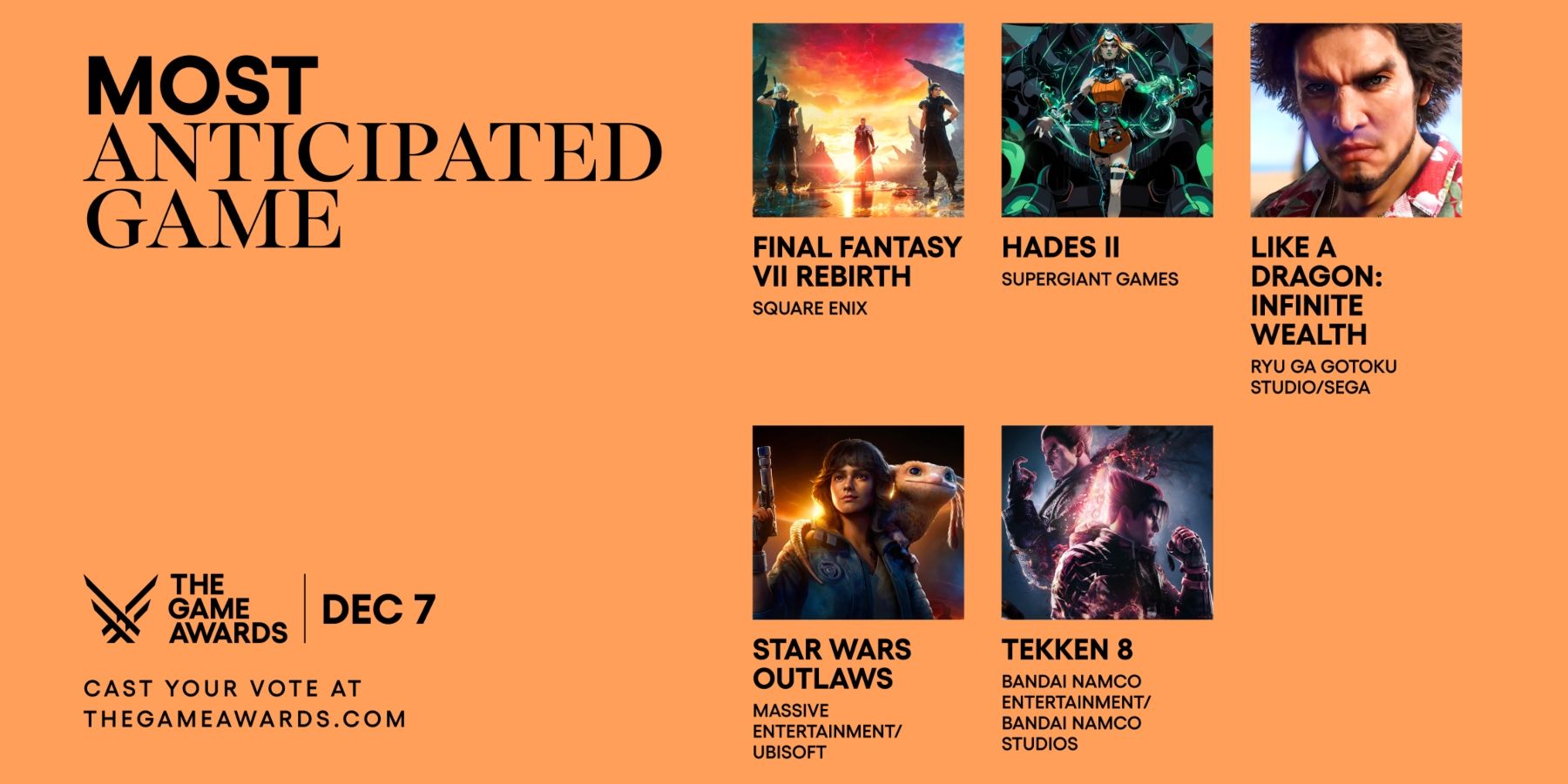This banner graphic, set against a striking orange background, serves as an advertisement for the Game Awards' "Most Anticipated Game" category, taking place on December 7th. Dominating the top left corner, bold black sans-serif and thin serif fonts spell out "Most Anticipated Game." Positioned at the bottom, the Game Awards logo is accompanied by a prompt to "cast your vote at thegameawards.com," displayed in small black text at the bottom left corner. The graphic features five square thumbnails of nominated games, each captioned with their title and production company. The top row showcases "Final Fantasy VII Rebirth" by Square Enix, "Hades II" by Supergiant Games, and "Like a Dragon Infinite Wealth" by Ryu Ga Gotoku Studio and Sega. The bottom row features "Star Wars Outlaws" by Massive Entertainment and Ubisoft, and "Tekken 8" by Bandai Namco Entertainment and Bandai Namco Studios.